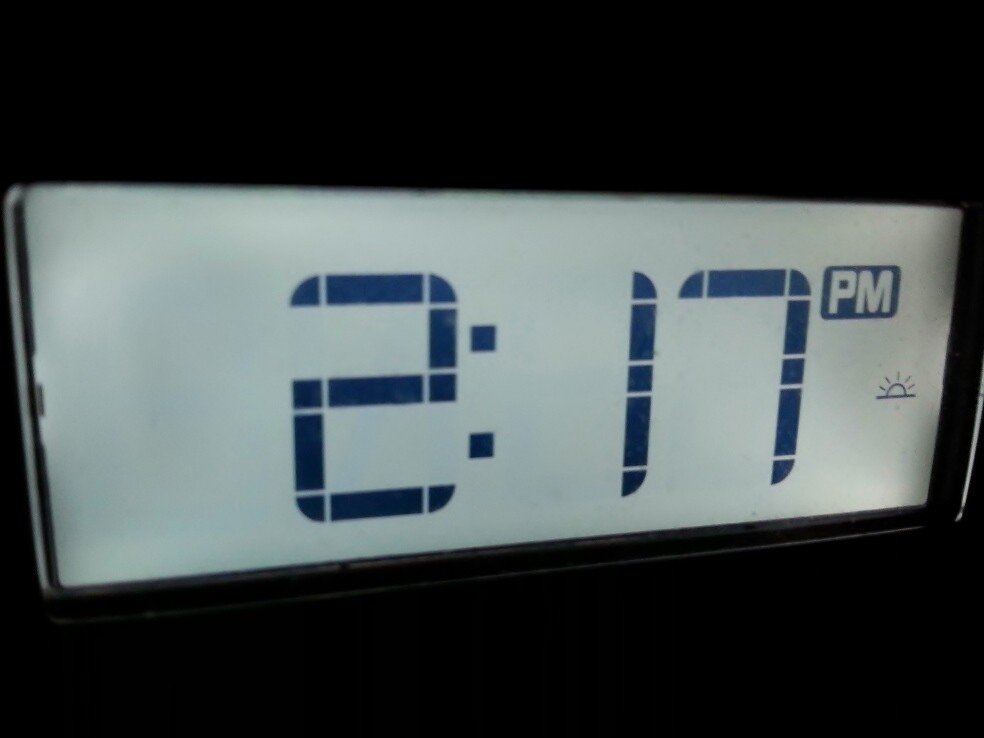This is a detailed photograph of a digital clock. The clock features a white face with dark blue digital numbers displaying the time as 2:17 p.m. Each number is composed of angular shapes, including rectangles and squares, giving the display a modern, geometric look. To the right of the time, there is a small icon of a sun, indicating daylight hours. To further clarify the time, the "p.m." designation appears in white lettering within a small blue square situated to the right of the "17." The clock's casing is black, and a beam of light illuminates the right side, enhancing its sleek design against the black background.